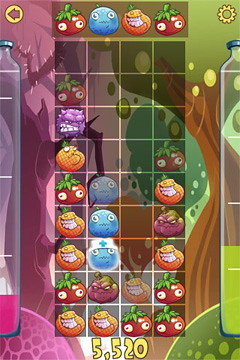The image is a screenshot of a mobile game captured in portrait orientation, evident from its tall and narrow frame which suggests its platform. The game interface features a back arrow icon at the top left corner, indicating a touch-based interaction which is characteristic of mobile games.

The game appears to be a matching puzzle game reminiscent of Tetris, organized into a grid comprising four columns and nine rows. The objective likely involves aligning or matching various quirky fruit characters. The distinctive fruits include apple or tomato-like figures with large white eyes, a blue fruit resembling a frightened blueberry, and an orange fruit character with a manic grin, each adding a whimsical element to the gameplay.

On the left side of the screen, there is a red bar designed to look like a bottle, and a similar green bar is situated on the right. These bars could potentially represent game metrics such as levels, scores, or remaining moves, adding another layer of engagement to the experience.